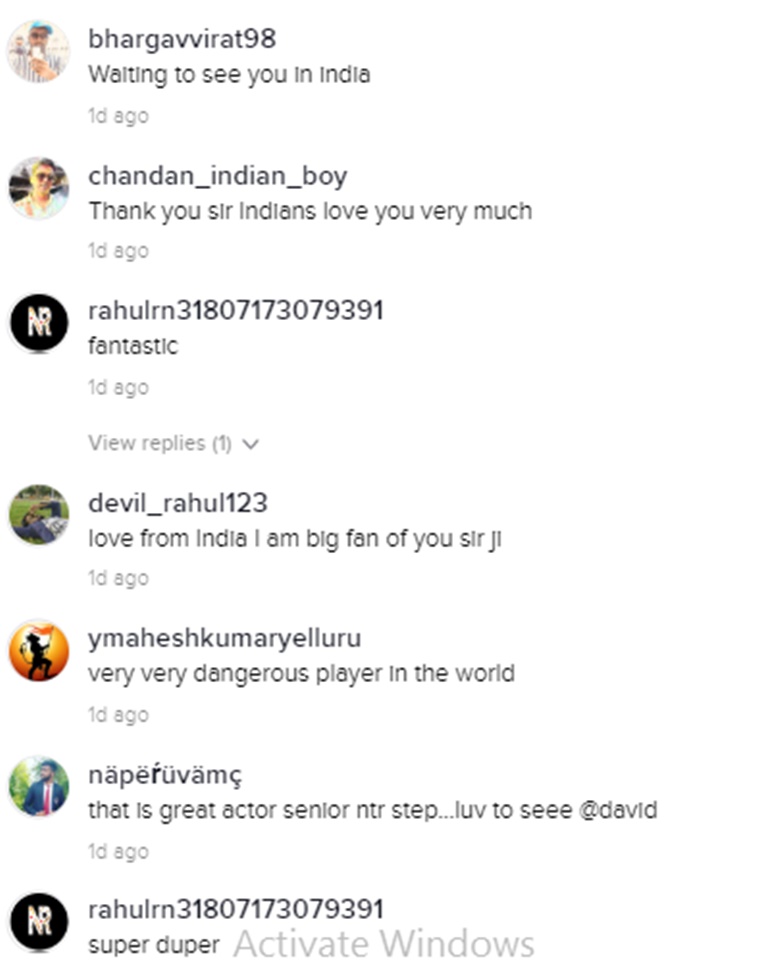Screenshot of a Chat Interface

This screenshot captures a set of interactions on a social media platform, likely Twitter, given the inclusion of user icons to the left of each comment and the format of usernames. The comments appear to be praise and expressions of admiration for an individual, potentially a celebrity or public figure, from various fans. The detailed comments are as follows:

1. **Bahar Gavirat 98**: "Waiting to see you in India." (Comment posted one day ago)
2. **Sean_done_Indian_boy**: "Thank you, sir. Indians love you very much." (Comment posted one day ago)
3. **Ra_here_LRN [followed by a long numeric string]**: "That's fantastic." (Comment posted one day ago, includes a hidden reply indicated by a dropdown menu labeled 'View replies.')
4. **Devil_Rahul123**: "Love from India. I am a big fan of you, sir." (Comment posted one day ago)
5. **Yam_hash_Kuma_yell Roo**: "Very dangerous, very very dangerous player in the world." (Comment posted one day ago)
6. **In_a_PERU V aMC [difficult to pronounce handle]**: "That is a great actor. Senior NTR... love to see [incomplete] David." (Comment posted one day ago)
7. **Rahul Rahul**: "Super duper." (Comment posted one day ago)

The image captures a diverse set of affections and accolades directed towards a central figure, emphasizing their popularity and the global nature of their fanbase.